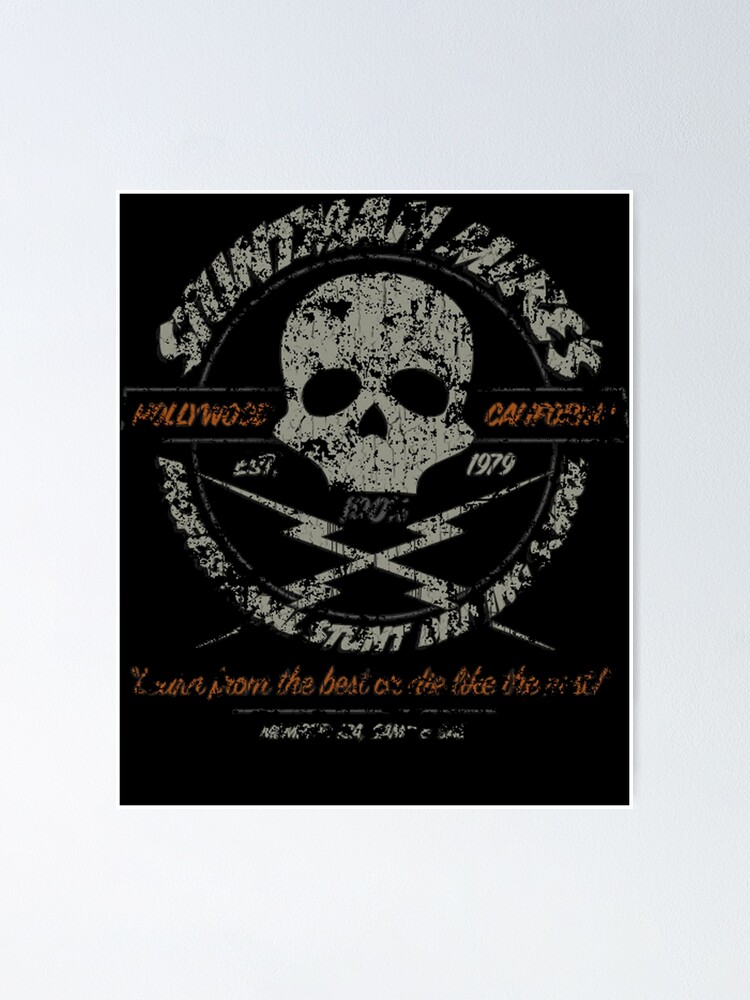This image depicts an old, weathered club poster with a black background and gray accents. The focal point of the poster is a partially visible human skull—displaying only the upper jaw—outlined in a worn graphic style. Flanking the skull are the words "Hollywood" on the left side and "California" on the right, with "EST 1979" positioned beneath them in orangey text that has significantly deteriorated. The skull is set against a backdrop featuring two lightning bolts crossed to form an X shape. At the bottom of the poster, there is text in goldish hues, partially discernible as saying something akin to "Stunt Prom: The Best Of or Die Like The Rest." The overall impression of the poster is reminiscent of an old, overly washed t-shirt, with its details being blurred and hard to read due to age and wear.